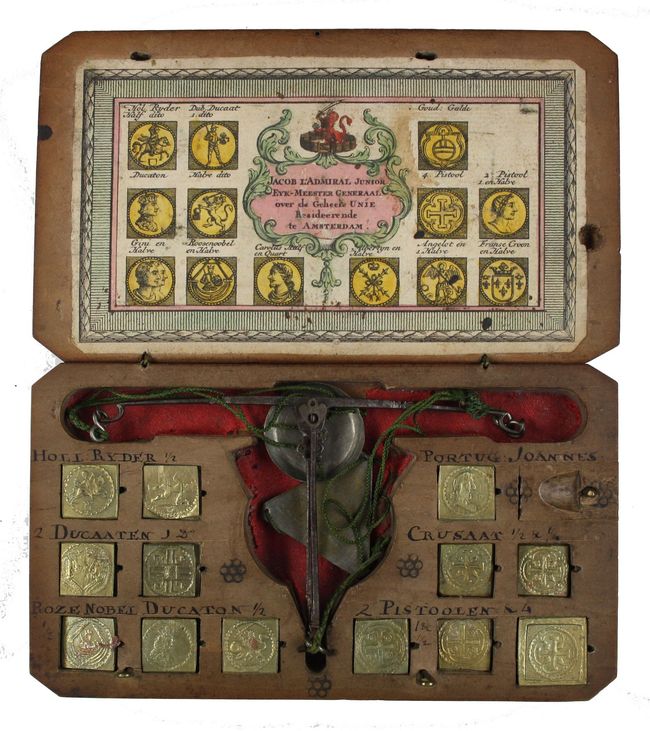The image depicts an extremely old, potentially 16th or 17th-century box, possibly of Spanish or Portuguese origin, with an open lid. The box, which may resemble a jewelry box but contains no jewelry, features intricate compartments and detailed labeling in a foreign language. The interior of the lid showcases a picture illustrating the box's contents, complete with labels, including various yellow squares with circles, faces, full-body figures, and horse riders. 

The main compartment appears lined with red felt and houses a number of gold squares—seven on the left and six on the right, totaling thirteen gold squares. These squares are likely not coins due to their shape. In the center of the box lies a mysterious black metal and possibly leather object resembling a bell or tool, adding to the box's mystical and medieval aesthetic. The overall design, filled with symbolism and depicting men, statues, and potential mythological imagery, evokes a sense of ancient, almost mystical or even satanic fortune-telling artifacts. This detailed box clearly holds a significant historical and perhaps mythical value, given its ornate craftsmanship and layered symbolism.